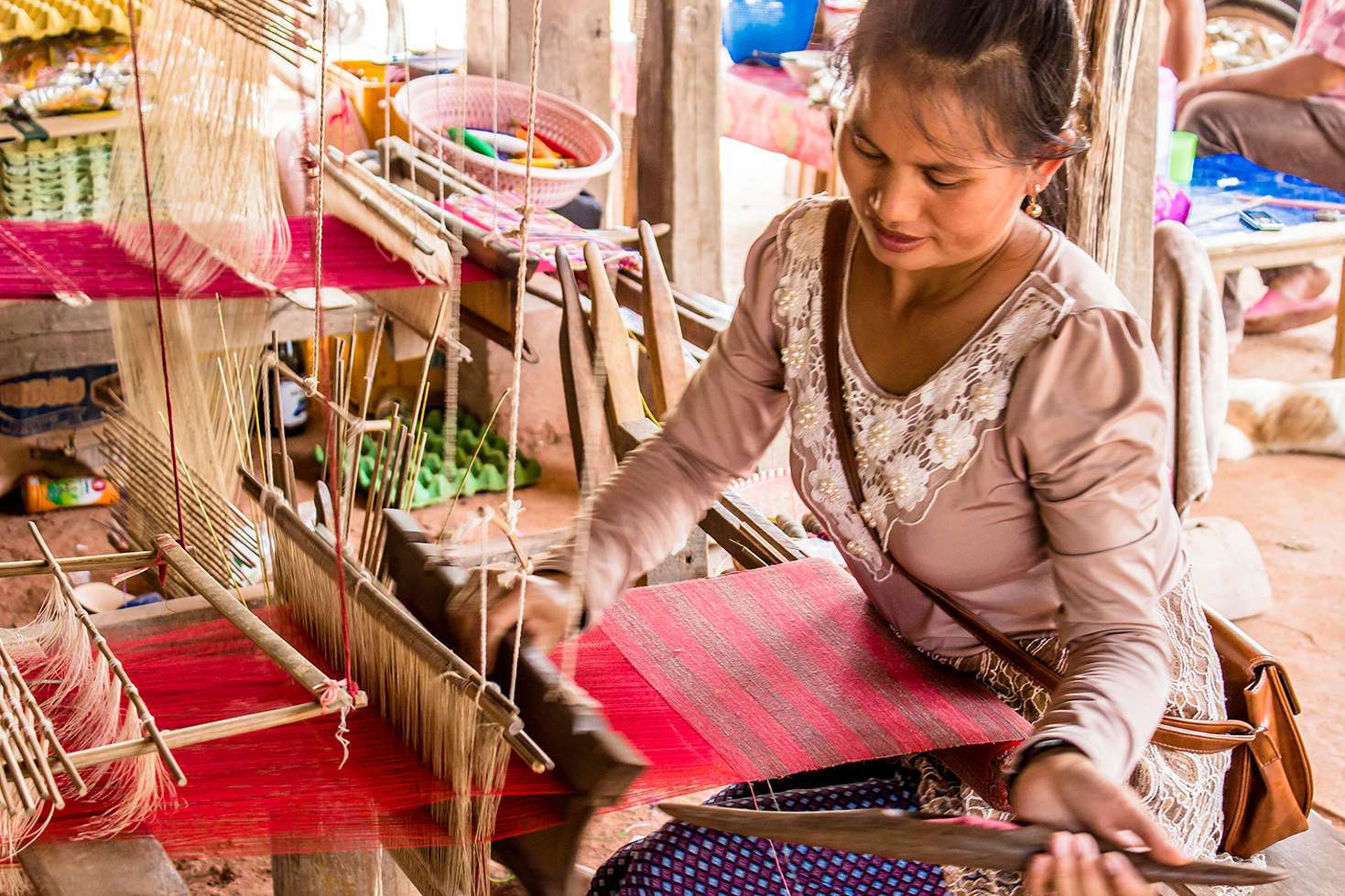In the vibrant setting of an outdoor Asian or Indian market, amidst the hustle and bustle of people sitting on stools in the background, a focused woman sits at an older-looking loom in the foreground. She is intricately weaving a fabric that features an alternating pattern of pink and dark red or rose and light brown stripes. Strands of yarn in various colors—green, white, orange, and yellow—are neatly arranged around her, alongside other looming tools and baskets to her right. The woman is dressed in a long-sleeved tan top with a delicately embroidered or doily-like collar, complementing her pulled-back brown hair and wispy bangs. Dark lipstick accentuates her focused expression. A brown purse-type bag, slung across her body and resting near her tailbone, completes her attire. With a weaving tool in her left hand, she skillfully manipulates the yarn strung over and above the loom, creating an exquisite piece of fabric.